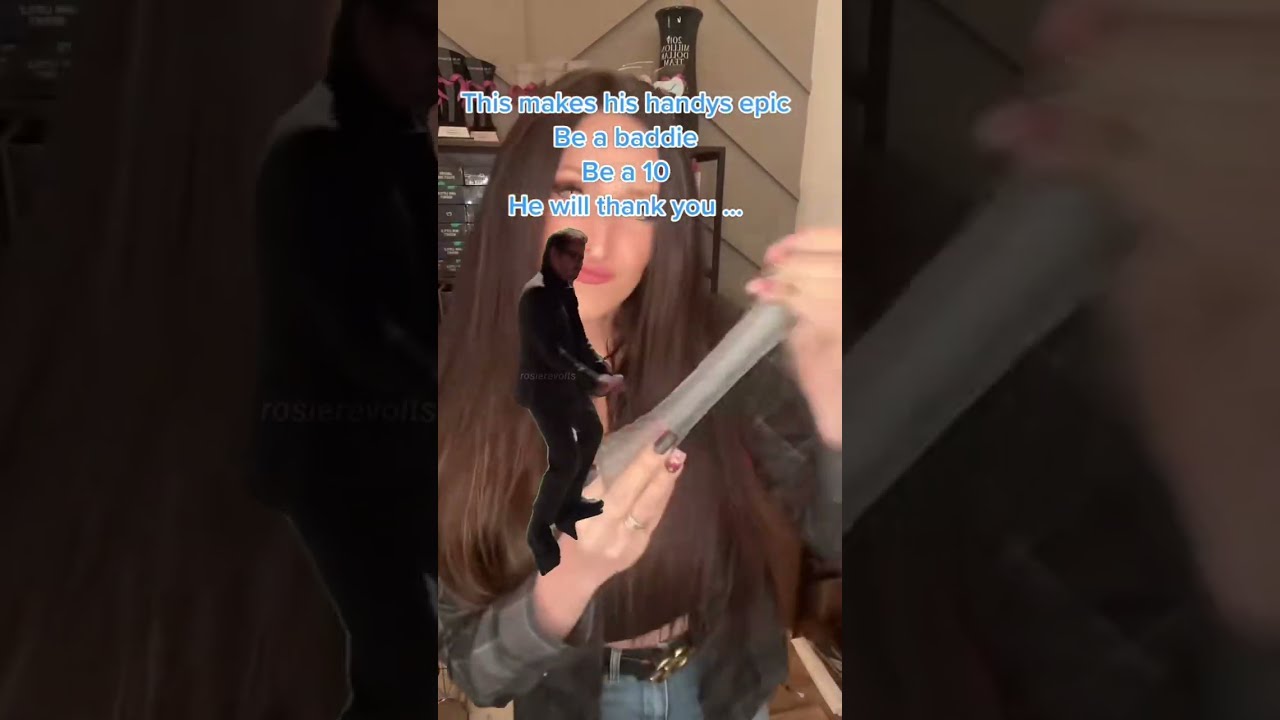The image is a horizontally rectangular collage featuring three separate panels. Each panel highlights different aspects of a central photograph of a woman, presumably taken in a vertical format resembling a TikTok still frame. The central image is clear and brightly lit, depicting a woman with long brown hair that reaches her chest. She is holding a mysterious cylindrical, silver or glass object with a murky white finish, using both hands—her right hand at the bottom and her left hand at the top. She is dressed in a brown shirt, blue jeans, and a black belt, with a plaid jacket partially visible on her. 

Overlaying the central image is a tiny 3D-rendered or photoshopped figure of a man in a black jacket, glasses, and dark pants. The man appears shadowed, directly in front of the woman’s hand holding the object, creating an unusual and unnatural effect. Nail polish is visible on her fingers, adding detail to her appearance. 

The text, in small, fuzzy blue font, is placed at the top center of the central panel, partially obscuring her eyes. It reads: "This makes his handies epic. Be a baddie. Be a ten. He will thank you." This text suggests some sexual innuendo. The left and right panels are darker and appear to be zoomed-in, cropped sections of the central image. The left panel shows just the lower part of her face and body profile against a brown background, while the right panel is a close-up of her left hand holding the object, with some blurred parts of her hair, arm, and background visible. Behind her, shelving and a wall are faintly visible, adding context to the setting.